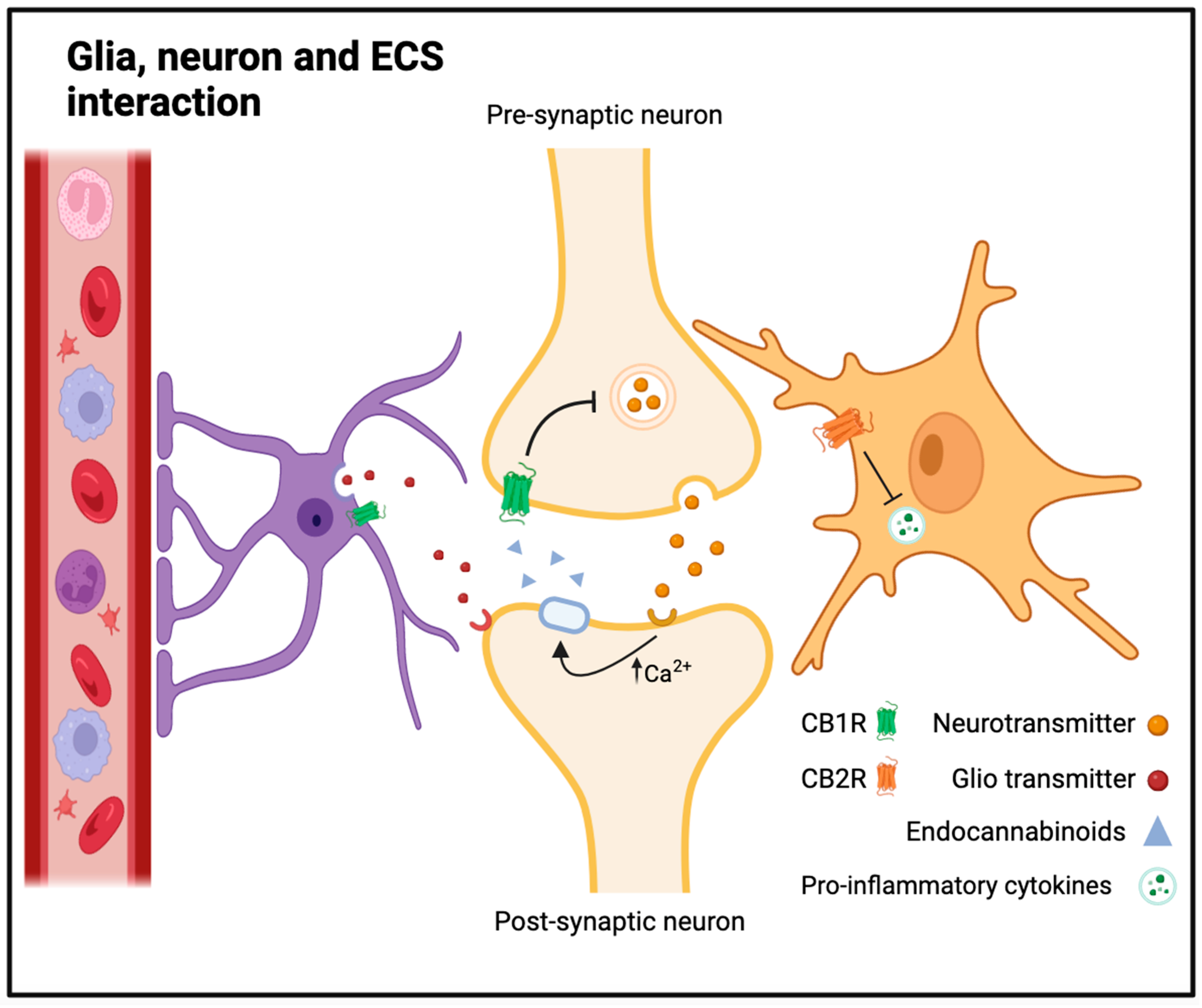This detailed medical diagram, set against a white background with a thin black border, illustrates the interaction between Glia, neurons, and the ECS. In the top left corner, large bold black text titles the image "GLIA, Neuron, and ECS Interaction." At the top center, "presynaptic neuron" is labeled, with "postsynaptic neuron" positioned at the bottom center. Between these, two bone-like structures curve towards each other, creating a visual of interconnected neurons.

To the left, an illustration resembling a blood vessel or vein contains red blood cells interspersed with other cellular forms. Attached to this vessel is a dark purple, alien-like structure with branching tentacles, featuring a central black dot akin to an eye.

On the right side of the diagram is a brown, amoeba-like blob with stubby branches extending from it. In the image's bottom right corner, a legend explains various particles floating around the neurons: yellow circles represent neurotransmitters, red circles symbolize gliotransmitters, blue triangles indicate endocannabinoids, and green dots signify pro-inflammatory cytokines.

This intricate depiction underscores the complex interactions within the neural and ECS systems, providing a comprehensive visual aid for understanding these biological processes.